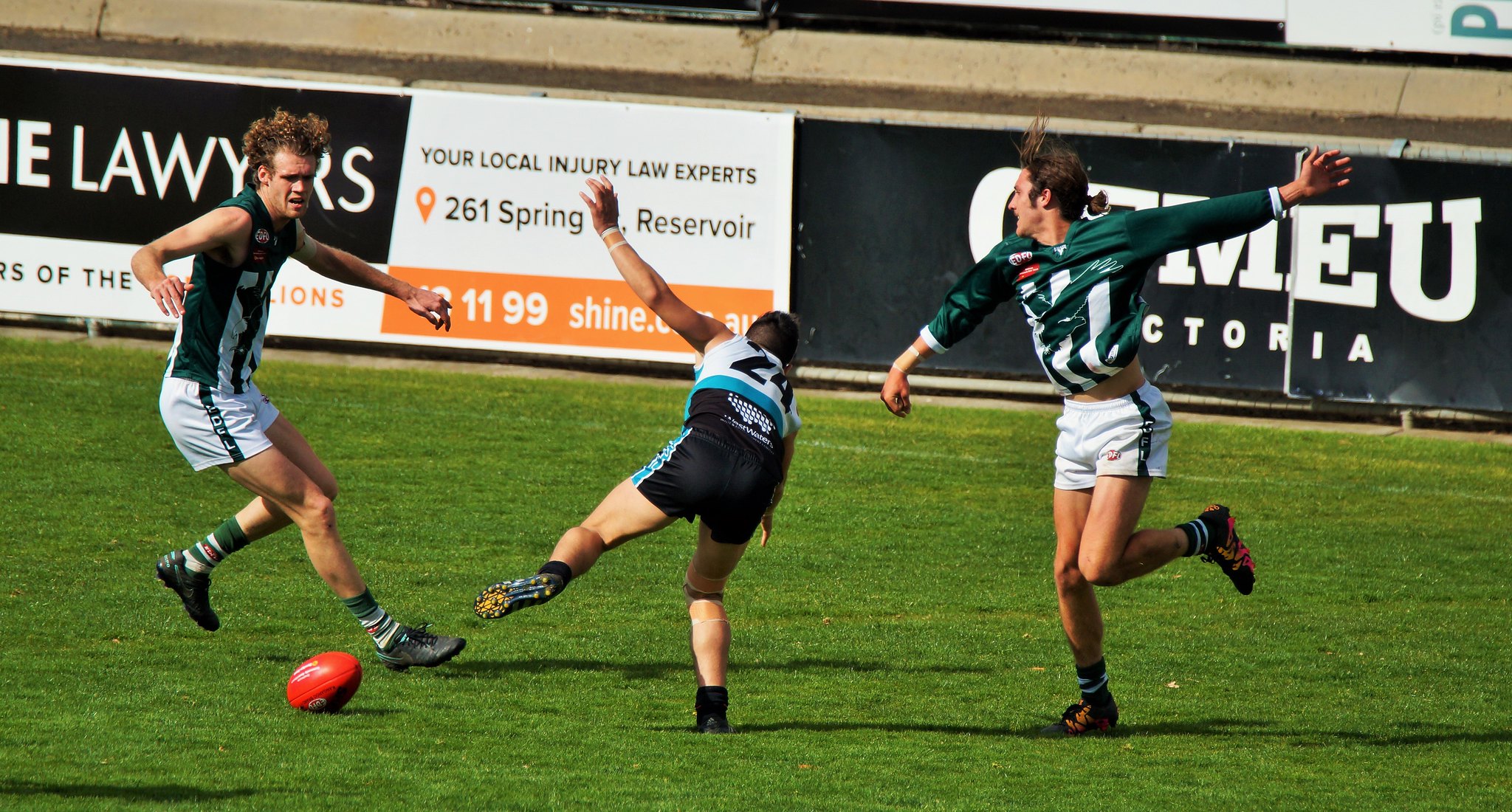This image captures an intense moment in what appears to be a rugby or Australian rules football match, set on a sunny day on a well-maintained, green grass pitch. Three players are in the thick of the action: two from the same team, wearing green jerseys with white symbols, white shorts, and green-and-white striped socks. The player on the right, sporting red shoes, has his left arm raised and right arm pointing down. His teammate on the left mirrors the uniform, with one arm extended and the other hanging down. Both players focus intently on a red rugby ball lying on the ground. Positioned between them, an opposing player clad in a white jersey with a blue belt and black shorts appears to be mid-fall, with one leg airborne and the other grounded, indicating a dynamic struggle for control. 

The background features a barricade adorned with various sponsor banners, including recognizable texts such as "lawyers in white on black," "your local injury law experts," and partial phrases like "MU Victoria." This suggests a well-supported match being held in a notable venue. The scene is vividly illuminated by daylight, enhancing the live-action feel of the photograph.